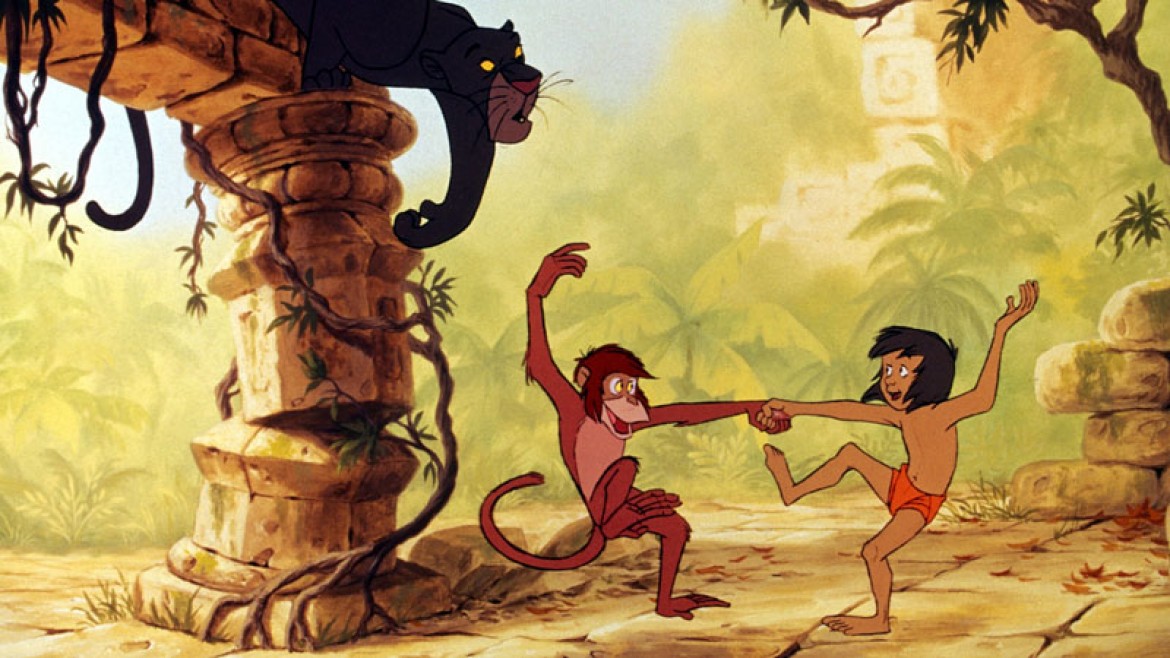In this animated scene reminiscent of a classic "Jungle Book" film, the setting is a vibrant jungle with a backdrop of green and yellow foliage, faded trees, and a vivid blue sky. In the center, a little boy with dark hair, clad in just shorts, joyfully dances hand-in-hand with a rusty orange-colored monkey. They strike a playful pose with one hand raised in the air, seemingly mid-song from the famous "I Wanna Be Like You" sequence. Surrounding them, a diverse array of jungle life adds to the dynamic atmosphere; you can spot various monkeys, including a baboon high up in the trees. On the left, silhouetted against the lush greenery, is a panther draped languidly over a shaped concrete pillar, its tail and one arm hanging down. Adding to the jungle's depth and texture are letter-like structures and stacked rocks. The entire scene is tinged with warm yellow and brown hues, evoking the earthy, untamed spirit of the jungle.